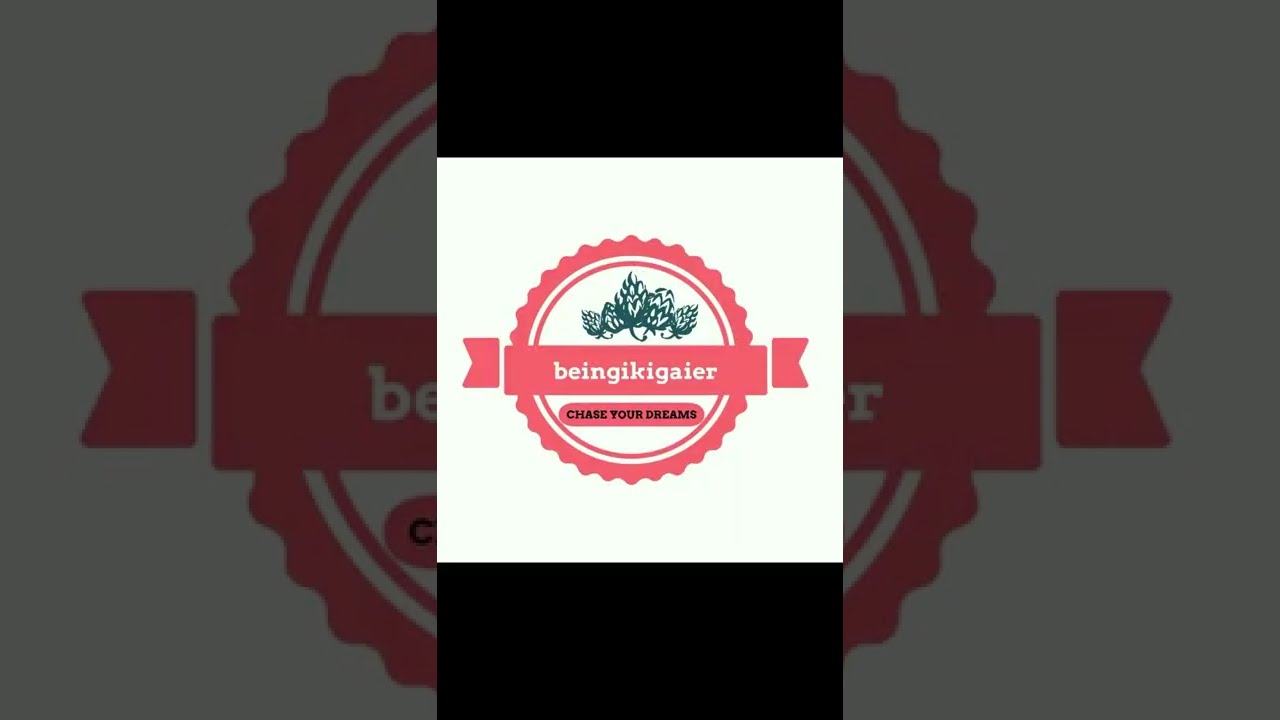This image is a business logo prominently featured in the center of a rectangular, landscape-oriented design segmented into three parts. The top and bottom segments display black bars, while the central segment features a white background with a detailed circular emblem.

The circular emblem comprises a red circle with a dark pink, spiky or cog-like edge. Within this circle, at the top, there is an illustration of dark green hop plants or floral elements in a clip-art style. Beneath these plants, a red horizontal banner spans across the circle, displaying the text "BEING I KAI GEHR" in white, lowercase letters with a fancy scroll-like design. Directly below the banner, another red bar contains the phrase "CHASE YOUR DREAMS" in black, all-capital letters.

The overall background outside the central segment is otherwise white, with larger, partially visible versions of the same logo design appearing to be faintly or obscured behind the main emblem. This layered design creates a focused central logo with a muted, repetitive pattern resembling the main emblem in the background.